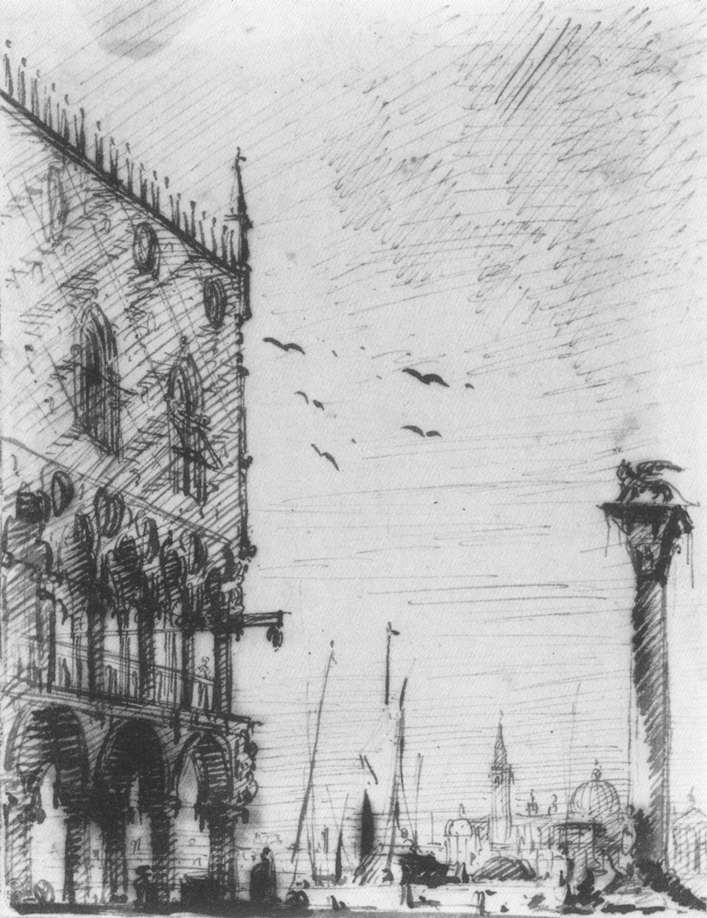The image depicts an abstract, black-and-white sketch that primarily uses ink and paper or pencil. The central focus is a large, ornate building on the left side, possibly resembling an apartment building with archways and columns on the first floor and elaborate windows on the upper floors. This building is detailed with a spiky rooftop and awnings over the windows. The background features a faintly sketched cityscape, with notable landmarks such as a domed building and what might be Big Ben, along with vague outlines that could be cranes or ship masts.

The sky is a broad expanse of hurried, sketchy lines, providing a light gray backdrop filled with black scribbles that suggest clouds and a dynamic group of birds, possibly seagulls, flying towards the left. On the right side of the image is a tall column crowned with a statue, which appears to be a lion with wings or perhaps an angel statuette. This column, placed on the bottom right corner, adds a vertical balance to the horizontally expansive scene. Overall, the drawing's abstract nature leaves room for interpretation, offering viewers a blend of recognizable architectural forms and imaginative artistry.